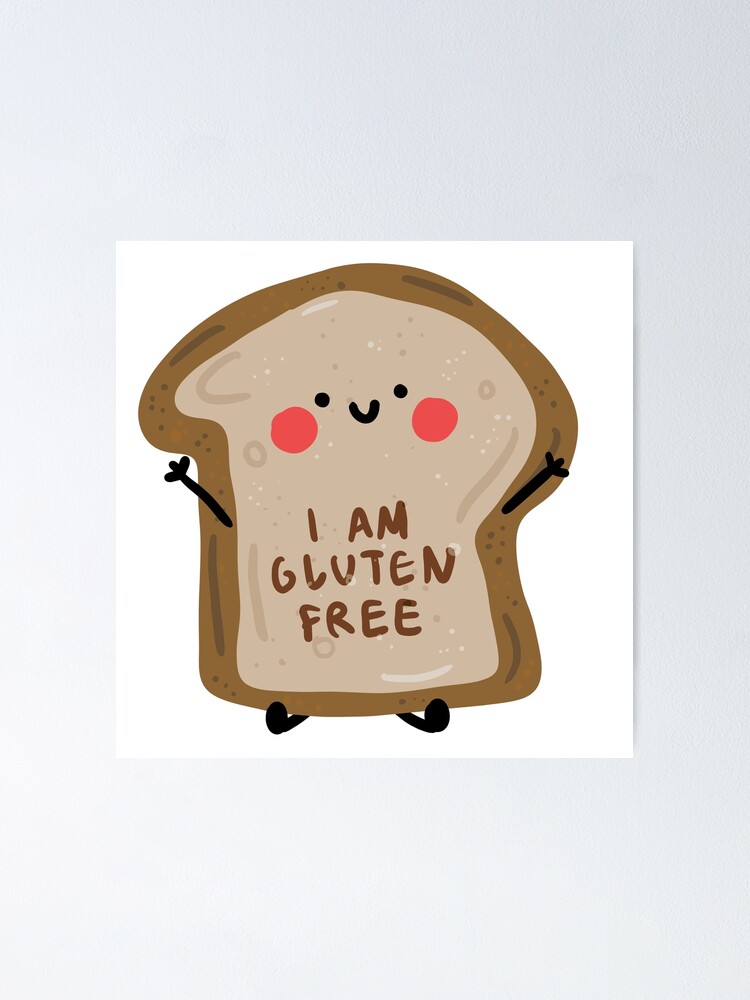This illustration features a cutesy, cartoon-like slice of whole wheat bread set against a plain white background framed by a light gray backdrop. With a dark brown crust and a lighter, tan interior, the bread is depicted with a simple, playful style that suggests it was painted with a basic paintbrush in Photoshop. The bread has a kawaii face, complete with two dot eyes, a U-shaped smile, and pink blush marks on its cheeks. It also sports black, stick-like arms and legs, with little Nike Chucks for feet. The phrase “I am gluten-free” is handwritten in brown across its stomach area, emphasizing the humor and charm of this happy, gluten-free illustration.